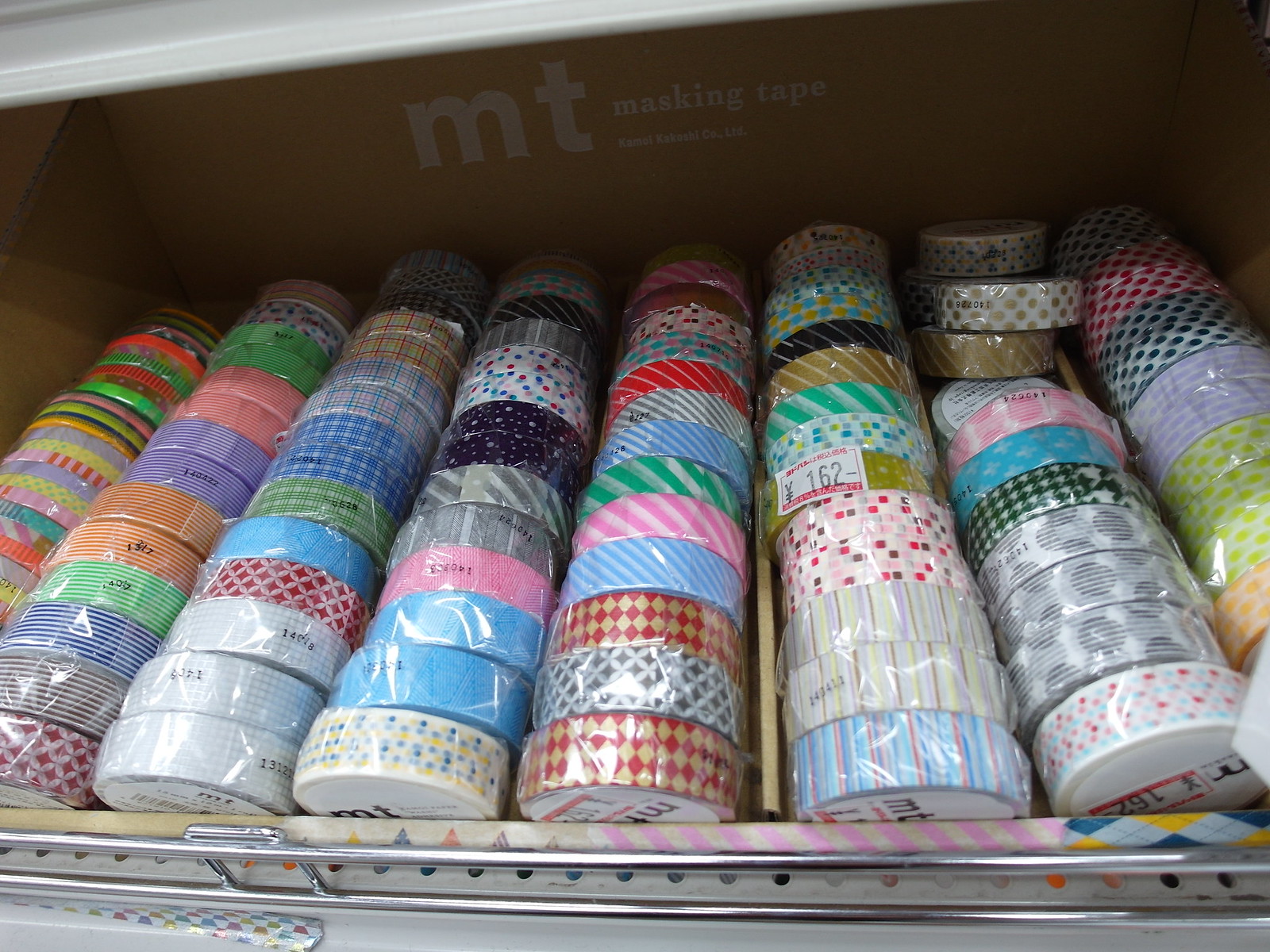The image captures a vibrant display inside a store, likely a craft or general store, showcasing a diverse assortment of masking tape rolls. The tapes, neatly arranged on a shelf inside a box, feature a label at the back reading "MT Masking Tape" along with the inscription "Camel Kokoschki Company Limited." Each roll of tape, encased in individual plastic coverings, boasts a unique pattern and color. The assortment includes stripes, floral designs, plaid patterns, polka dots, checkers, and diamond shapes in various hues such as blue, white, green, pink, and red. The rolls, organized into approximately eight rows with 10 to 15 rolls per row, offer a striking visual of multicolored and patterned masking tapes, suggesting a rich variety for any creative or decorative project.